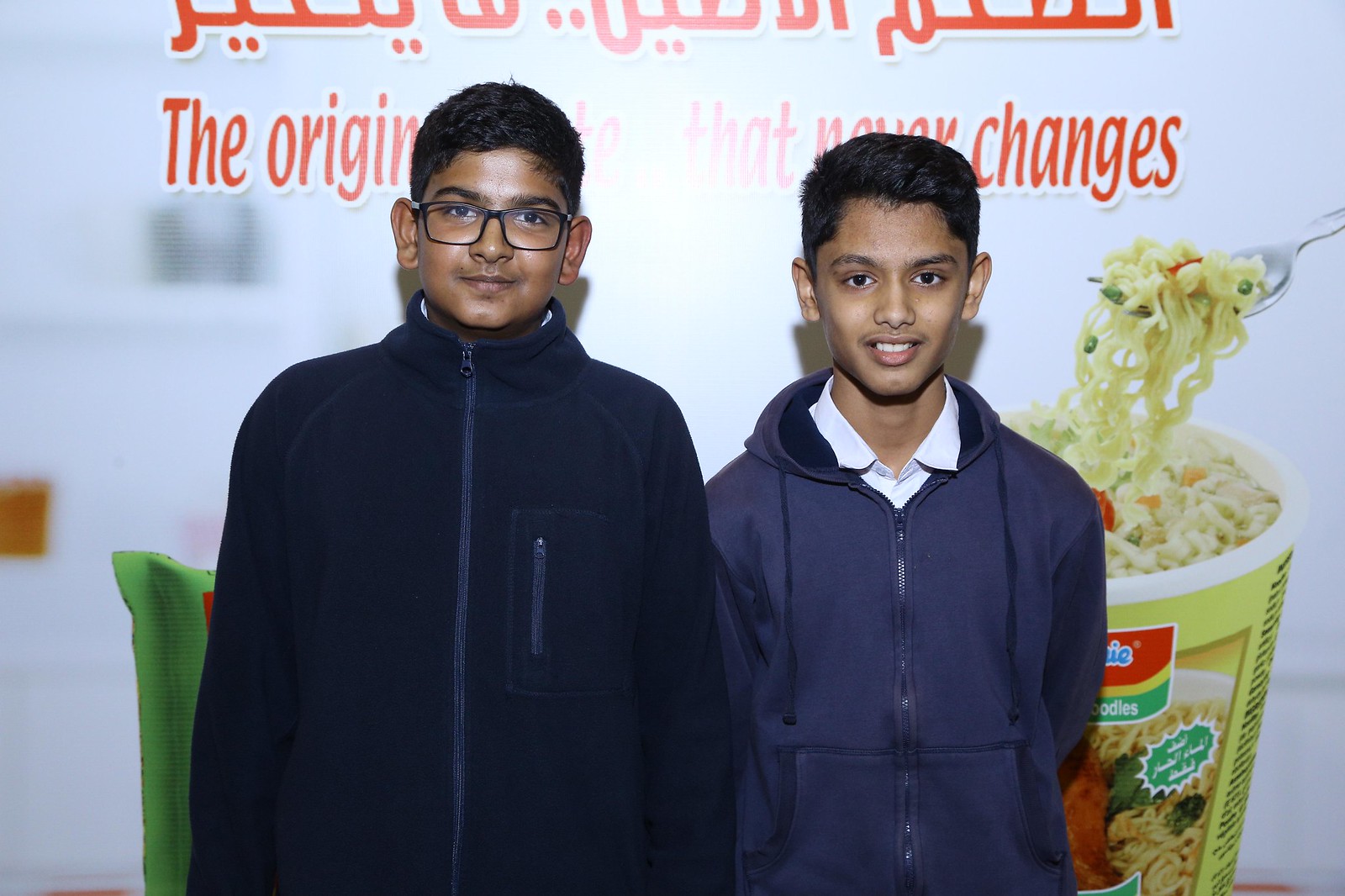The photograph captures two young Indian boys standing shoulder to shoulder against a backdrop featuring an advertisement. The boy on the left is taller and dressed in a navy blue jacket with a high collar and black-framed glasses. He has short black hair and an expressionless face. The boy on the right is slightly shorter, with a more pronounced square jawline and similarly short black hair. He is wearing a white collared shirt underneath a slightly lighter navy blue jacket that is unzipped, revealing the shirt's collar. Both boys are positioned in front of an ad, which prominently displays a green cup of ramen noodles being lifted by a fork. The cup features orange lettering, partially obscured but reading "noodles." Above the boys' heads, the text "The original something that never changes" can be partially read in English, with additional writing in Hindi or another Indian language cut off at the top of the frame. The setup suggests they are standing in front of a promotional banner for a ramen noodle dish.